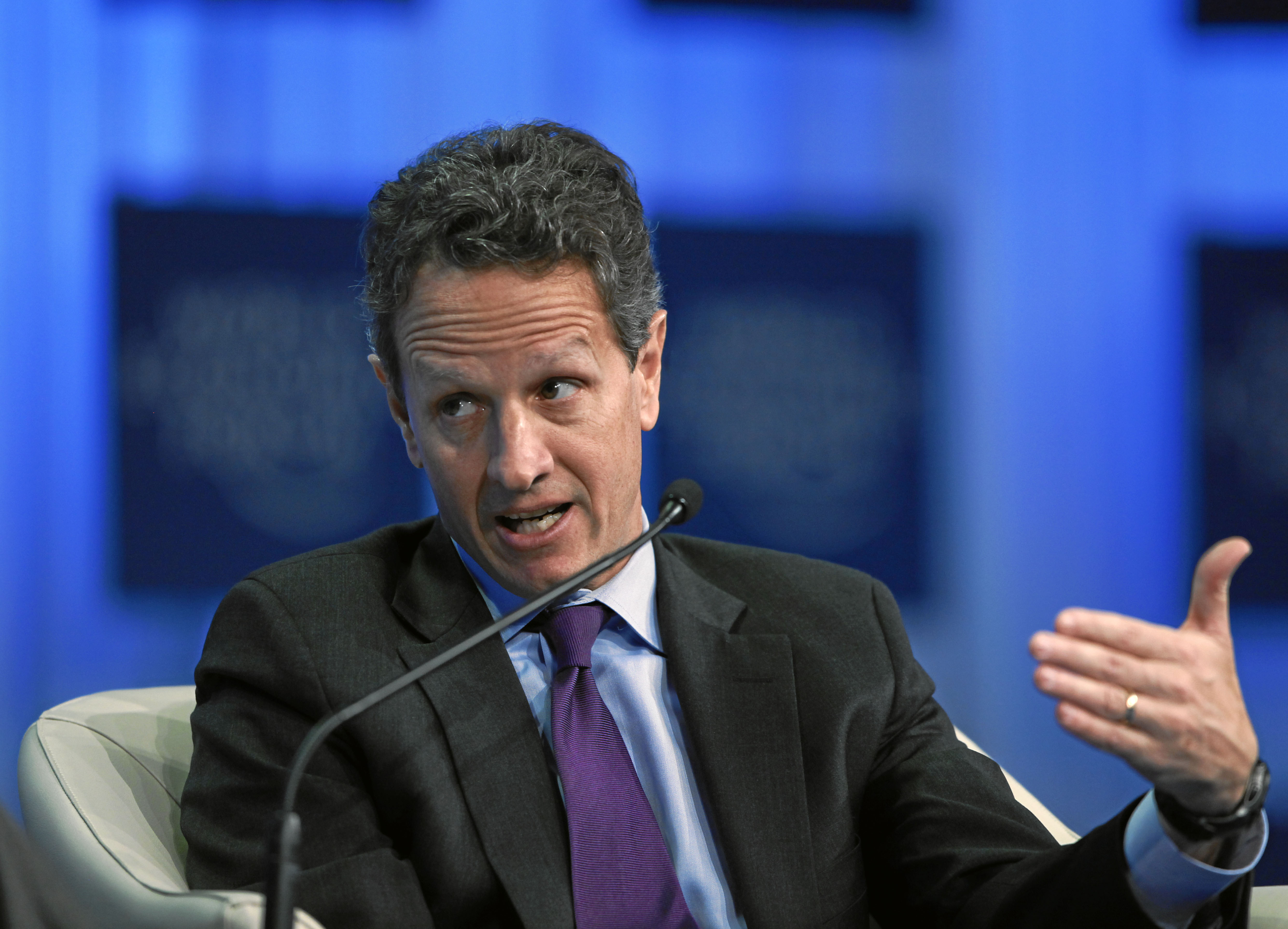The photograph captures a white male, possibly a famous politician, deeply engaged in a heated discussion at an event. He is seated in a white or light beige cushioned chair, wearing a dark black suit paired with a light blue shirt and a purple tie. A wedding band is visible on his left hand, which is raised to his chest level as he gestures animatedly, and a watch adorns his left wrist. His head is tilted slightly towards his right shoulder as he looks to the left, speaking into a long, thin black microphone in front of him. The backdrop comprises a bright blue wall adorned with blurred darker blue signs or screens, possibly containing some graphics or text, which adds depth to the scene while keeping the focus on the speaker.